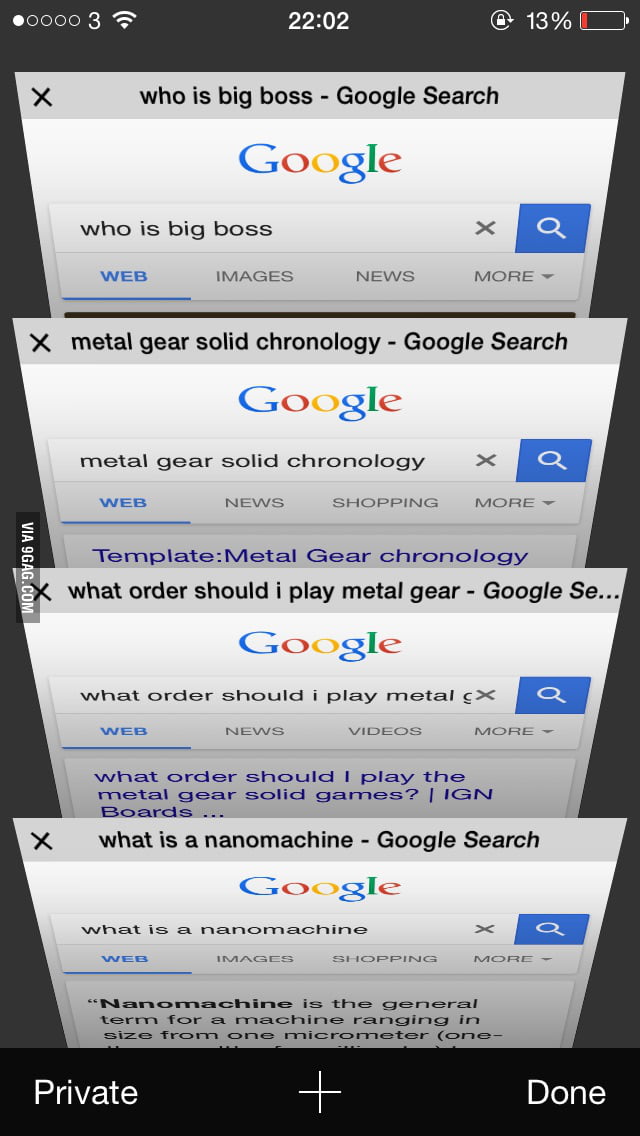The image depicts a smartphone screen displaying a sequence of four Google search cards, all against a black background. Each card appears as though layered like documents in a file stack. 

- The **first card** displays a Google search with the query "Who is Big Boss" visible inside the search bar, accompanied by the Google logo.
- The **second card** contains the search term "Metal Gear Solid Chronology". Beneath this, one of the search results reads "Template: Metal Gear Chronology".
- The **third card** shows the search query "What order should I play Metal Gear", and a specific result from IGN titled "What order should I play the Metal Gear Solid games?" is visible below the search bar.
- The **fourth and final card** features the query "What is a nano machine".

This screenshot illustrates an individual's detailed inquiry into the Metal Gear Solid video game series, starting from identifying key characters to understanding the gameplay sequence and specific in-game elements.